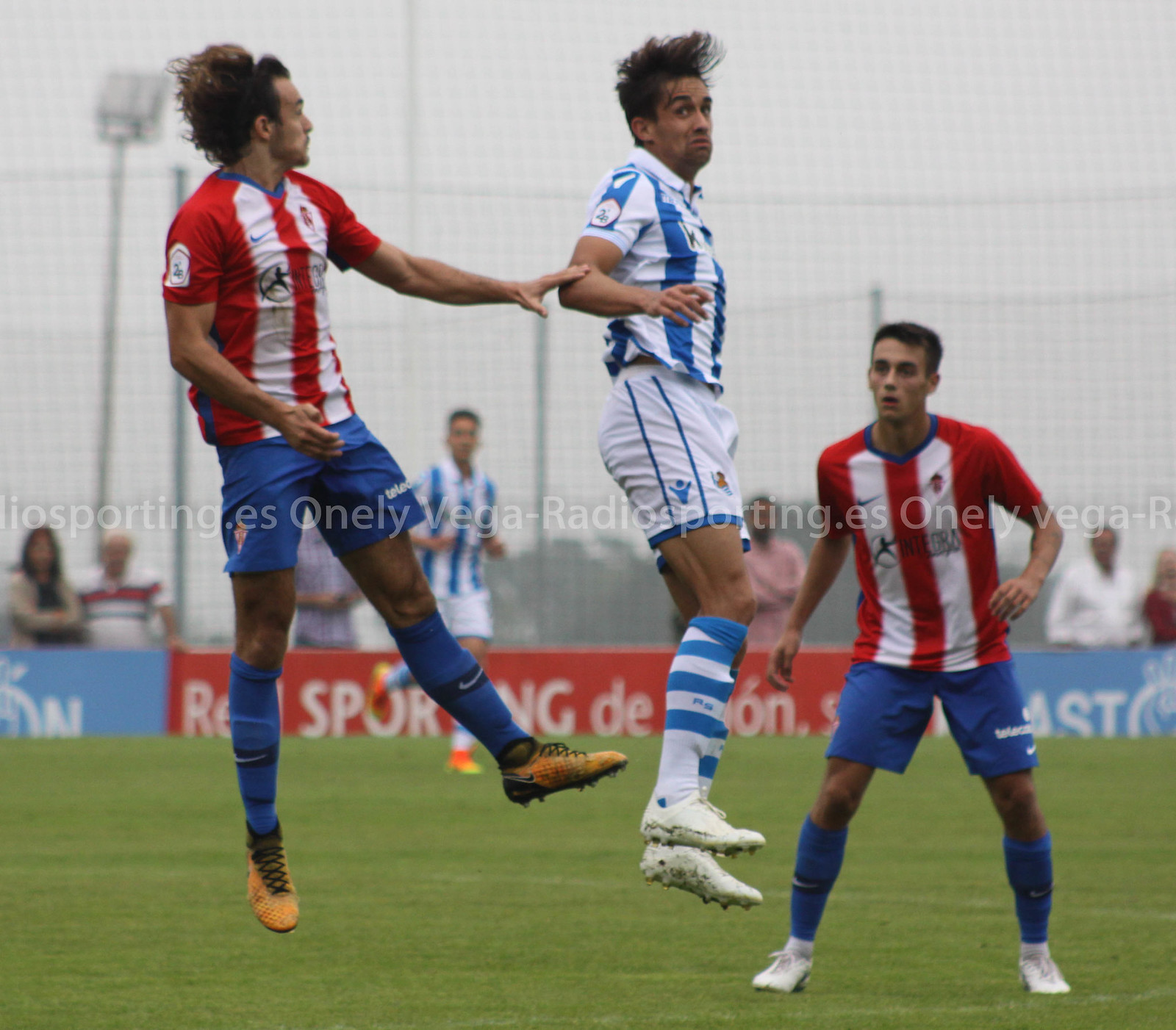The image captures an intense moment in a soccer game on a dark green grass field. Central to the scene, two players from opposing teams are caught midair, seemingly vying for the ball. The player in blue and white, who sports white cleats, striped blue and white socks, and a matching uniform, is leaping prominently. To his left, another airborne player—wearing orange cleats, blue socks, blue shorts, and a red and white vertical striped jersey—has his hand on the first player's arm. To the right of the central player, a teammate of the player in red and white stands ready; he is outfitted similarly with white cleats instead. Behind them, a referee is visible, along with indistinct bystanders standing behind a netting or fence. Another player in a blue and white uniform with white shorts and orange cleats can also be seen in the background. The image bears a watermark that is partly legible and appears to be in Spanish.